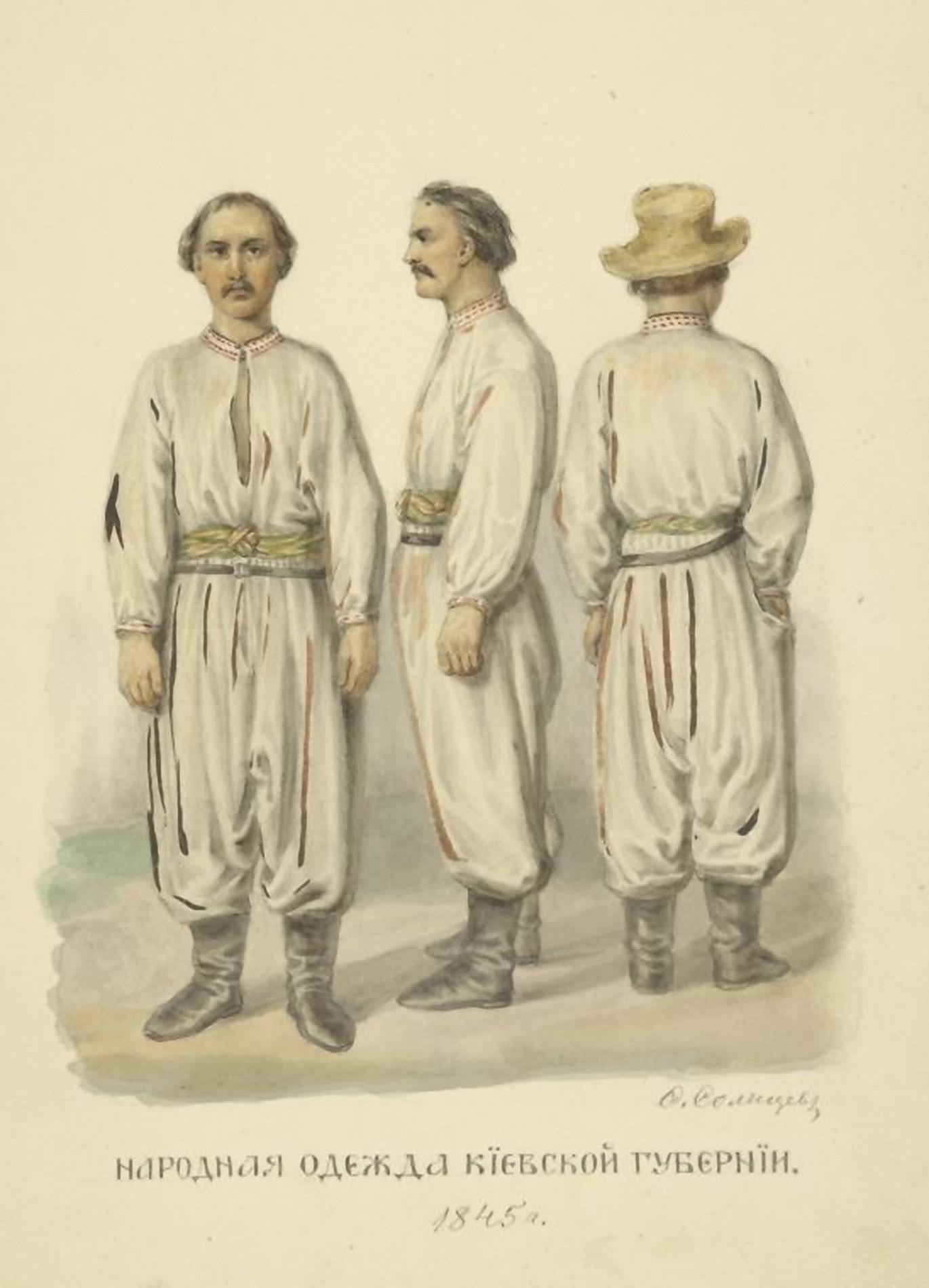This vintage color illustration, dated 1845, depicts an older gentleman portrayed from three different angles on an off-white, aged paper. The man, most likely the same individual shown in three positions, has short black hair, a mustache, and is balding. He is dressed in a traditional loose-fitting white pantsuit adorned with decorative embroidery around the waist and neck, and the pants are tucked into calf-length black boots. Notably, he wears two belts: a thin black one and a knotted gold rope. 

In the leftmost position, he faces forward without a hat. The middle figure presents his profile facing left, also hatless. The rightmost figure shows his back turned to the viewer, now wearing a brown, wide-brimmed hat. At the bottom of the illustration, there is a line of non-English text, possibly in Russian or Greek characters, along with the artist’s partial signature starting with "O" in a cursive script.